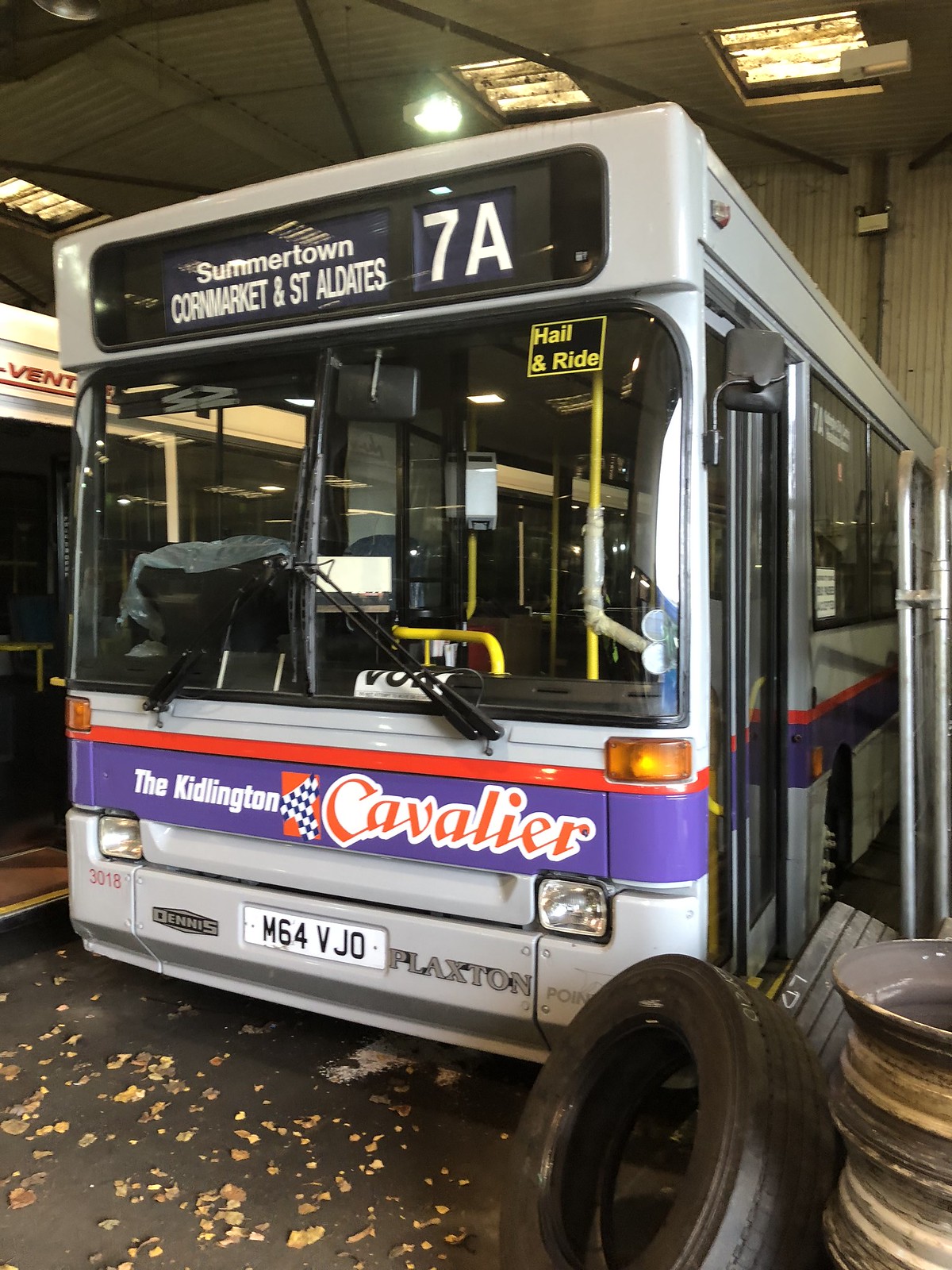This vertically aligned image depicts the front end of a city bus situated under a covered area. The bus features a white upper section with a digital display indicating its route to "Summertown, Cornmarket, and St. Aldates," alongside the code "7A" in white print. Below this digital screen, a yellow "Hail and Ride" sign is visible on the upper part of the windshield. The front of the bus showcases a blue and white color scheme with the inscription "Kidlington Cavalier" in white and red print against a blue background.

Notably, the license plate reads "M64 BJO," flanked by the names "Dennis" on the left and "Plaxton" on the right. The door on the right side of the bus (visible on the left side of the image) is open, and yellow bars are evident inside the bus. The driver’s position on the right-hand side underscores its operation in England. 

In the lower right-hand corner of the image, there are several wheel rims stacked atop one another with one or two tires leaning against them. Scattered leaves are visible on the street in front of the bus.